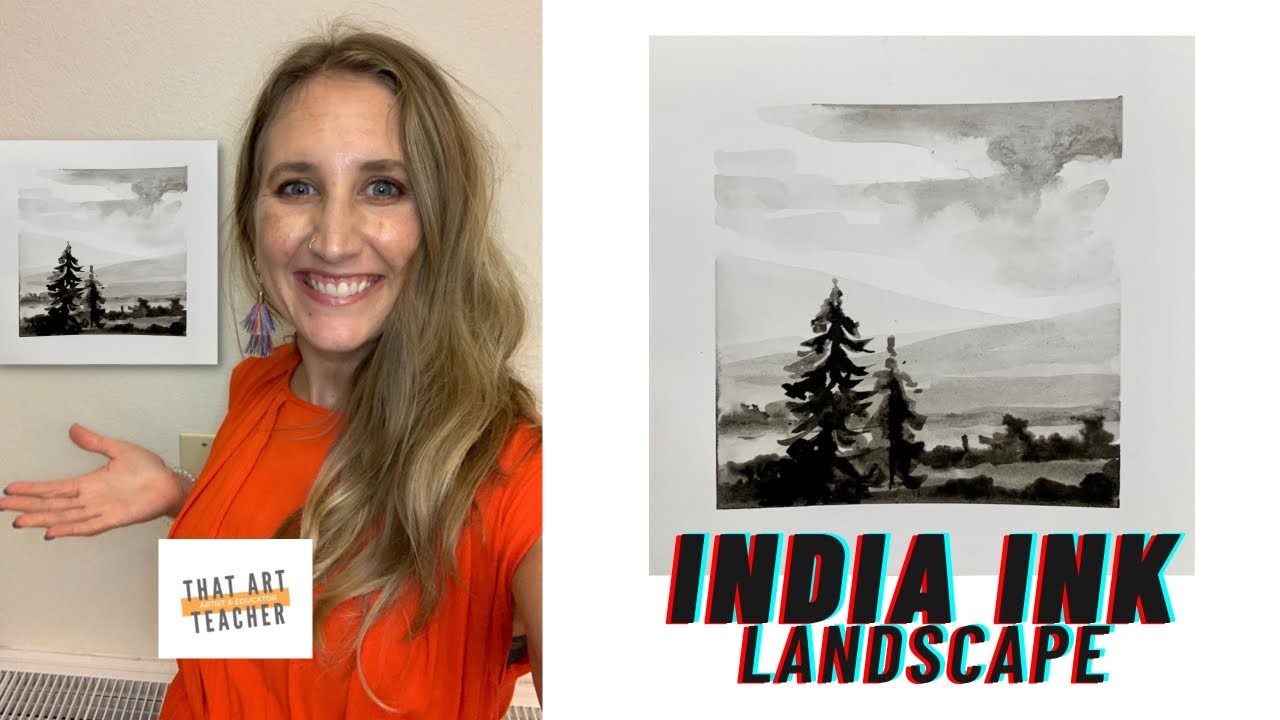The image features two side-by-side photographs. On the left, a young Caucasian woman with messy blonde hair, blue eyes, and a red blouse is captured from waist to mid-stomach up, looking directly at the camera with a smile. She stands indoors, in front of a light tan wall, next to a black-and-white artwork depicting a landscape with trees. Her left arm extends forward off-screen while her left hand is raised to chest level with the palm facing up. A small white square in the foreground, near her waist, reads "That Art Teacher." Behind her, the wall-mounted artwork is displayed with two tall pine trees and mountains in the background. On the right side of the image is an enlarged, detailed view of this same black-and-white artwork, titled "India Ink Landscape," showcasing a detailed ink representation of the natural scene. The photograph on the left is in portrait orientation, while the entire image is in landscape orientation, emphasizing the continuity and detail of the displayed artwork. The colors prominent in the image include orangeish red, orange, white, tan, blonde, blue, and black, with a clear focus on the black-and-white artistic elements.